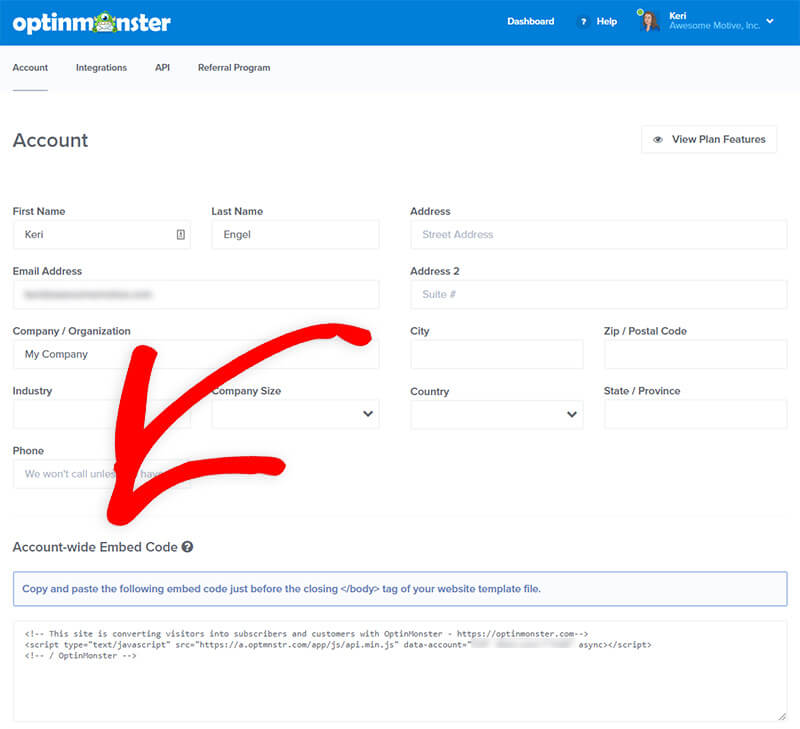The header of the website features a blue background on the top and white on the left-hand side. In the blue section, the word "DASHBOARD" is displayed in white. A blue circle with a white question mark is labeled "Help," while a green circle presents a blurry avatar, likely depicting a female character with fair skin, brown hair, and a blue shirt. Next to this avatar is the name "Keri," followed by "Motive, Inc."

The main content is displayed on a white background. At the top, underlined in black, are various sections: "Account," "Integrations," "API," and "Referral Program." Below these sections, there is a detailed account information form. The form fields include:

- First Name: Keri
- Last Name: Angle
- Address: "Free Address" in gray
- Email Address: Blurred out
- Company: "My Company"
- Organization: Not filled
- Industry: Not filled
- Company Size: Not filled
- City: Not filled
- Country: Not filled
- Zip Code/Postal Code: Not filled
- State/Province: Not filled
- Address Line 2: Suite Number not filled
- Phone Number: A red arrow covers this part, pointing down to the last section.

The last section lists account-wide settings, followed by an embed code area, indicated by a gray circle with a white question mark inside.